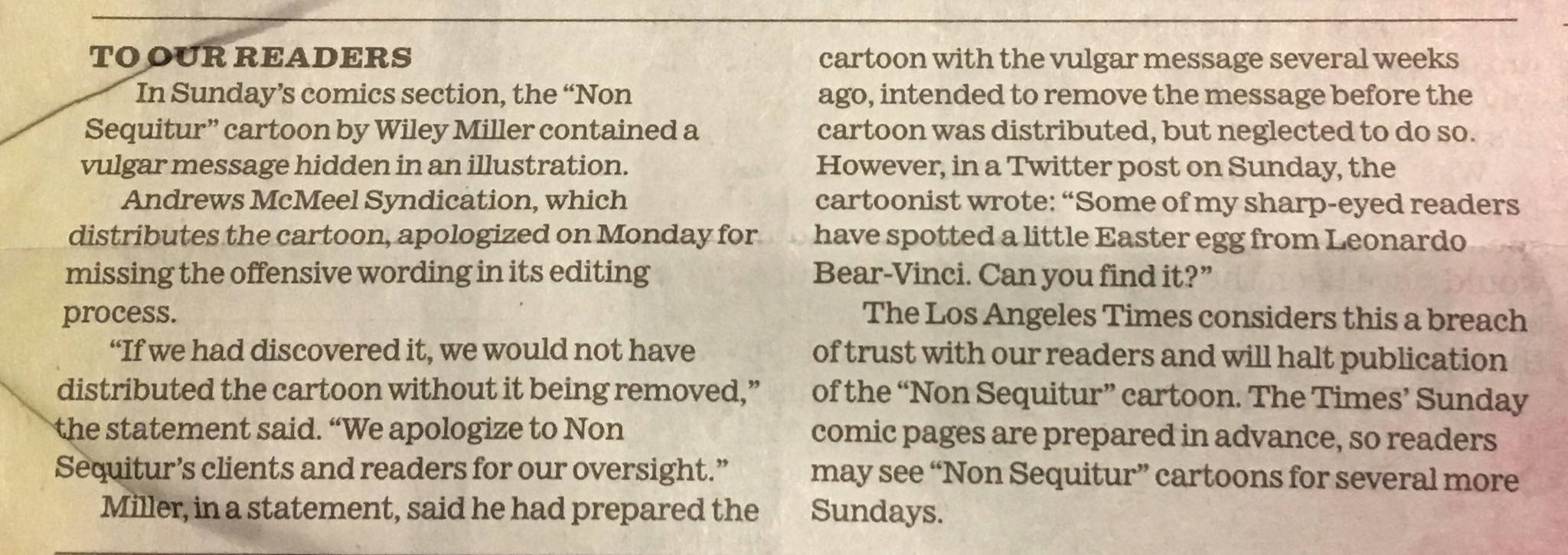The image is a photograph of a small, aged newspaper article with some browning and folds on the left side. The headline of the article reads "To Our Readers" in a bold black font. The article addresses a controversy involving the non sequitur cartoon by Wiley Miller, which contained a hidden vulgar message in an illustration in Sunday's comic section. Andrews McMeel Syndication, the distributor of the cartoon, issued an apology on Monday for not catching the offensive wording during the editing process. The statement emphasized that had the message been discovered, the cartoon would not have been distributed unchanged. Wiley Miller, the cartoonist, explained that he had intended to remove the message before distribution but neglected to do so. Complicating the matter, Miller had even hinted at the hidden message in a Twitter post, challenging readers to find an Easter egg from "Leonardo Bervinchi." The Los Angeles Times views this lapse as a breach of trust and has decided to halt the publication of the non sequitur cartoon. However, due to advance preparation of the Sunday comic pages, the newspaper noted that readers might still see non sequitur cartoons for several upcoming Sundays.